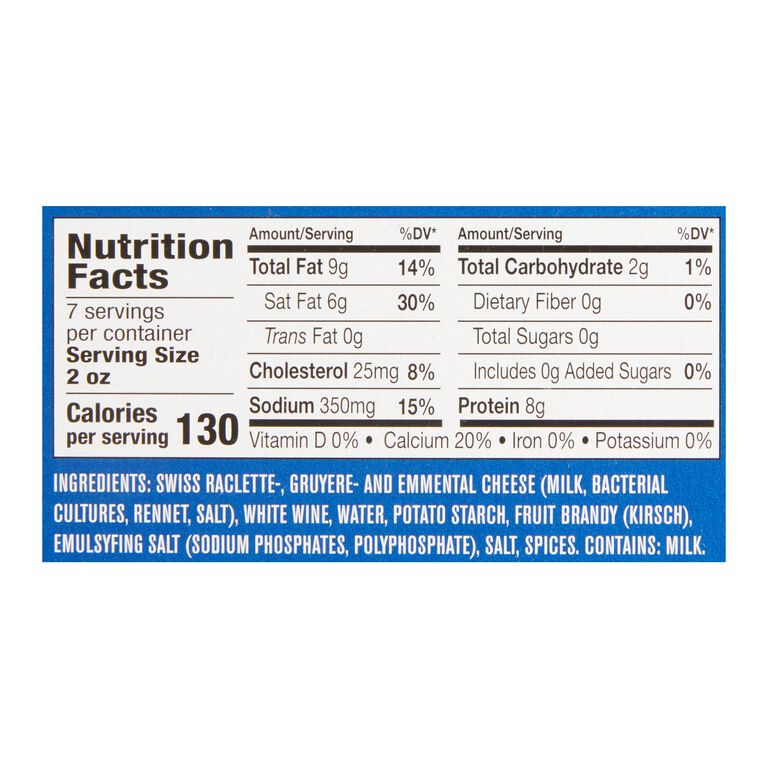This image displays a Nutrition Facts label on a blue background with white and black text, likely from the back of a box or bottle. It indicates that there are 7 servings per container, with each serving size being 2 ounces. Each serving contains 130 calories, 9 grams of total fat (14% DV), 6 grams of saturated fat (30% DV), 0 grams of trans fat, 25 milligrams of cholesterol (8% DV), and 350 milligrams of sodium (15% DV). Additionally, it lists 2 grams of total carbohydrates (1% DV), 0 grams of dietary fiber, 0 grams of total sugars with no added sugars, and 8 grams of protein. Nutrient information also includes 0% daily values for Vitamin D, iron, and potassium, but a 20% daily value of calcium. The ingredients listed are Swiss raclette, Gruyere and Emmental cheese, white wine, water, potato starch, fruit brandy, emulsifying salts, and spices, and it mentions that the product contains milk.